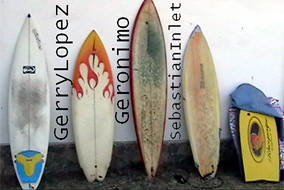The image depicts an outdoor scene featuring five well-used surfboards leaning against a white-painted stone wall. The surfboards, arranged on a gray stone pavement, display a variety of wear and colors. The first surfboard is primarily white with a worn spot in the middle, featuring a small blue area with a yellow moose head symbol at the bottom. The second surfboard is white with a splash of dark orange at the tip. The third and fourth surfboards are so worn that their original colors are barely distinguishable, though faded red markings are visible. The fifth surfboard is notably smaller, bright yellow, suggesting it might either be a shortboard or a broken piece. Alongside the surfboards are a couple of blue and yellow boogie boards. In the background, vertically spaced between the surfboards, is black lettering on the wall reading "Jerry Lopez, Geronimo, Sebastian Inlet." Additionally, a blue cover rests atop the yellow boogie board on the far right, completing the arrangement.